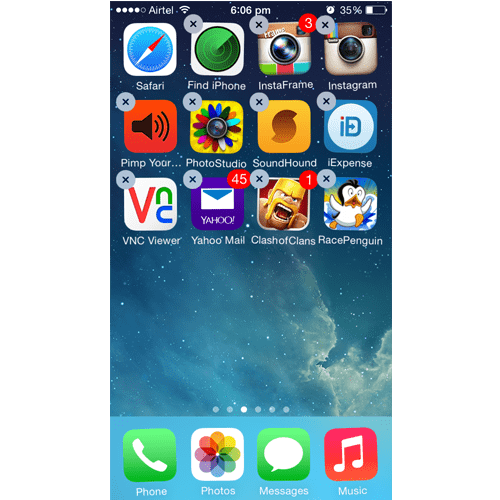A vertical screenshot of a smartphone home screen, commonly seen on devices like an iPhone or Android, is depicted with intricate details. It shows the status bar symbols at the very top: four out of five circles filled, indicating signal strength, and a blank one representing a missing quintile. The carrier name "Airtel," a Wi-Fi symbol, and the current time "6:06 p.m." are displayed next to battery information showing 35% power. The battery icon itself appears significantly depleted. 

The wallpaper exhibits a gradient background transitioning from blue at the bottom to black at the top, with subtle clouds and twinkling stars, evoking a serene twilight ambiance.

The home screen layout includes three rows of apps, each containing four icons. 

**First Row (left to right):**
1. **Safari**: A white square with a red and gray compass icon, the red arrow pointing northeast.
2. **Find iPhone**: A white square featuring a green radar.
3. **Instaframe**: A camera icon on a dark background with a red notification bubble displaying the number '3.'
4. **Instagram**: A camera icon on a gray circle with a black 'X' marker.

**Second Row (left to right):**
1. **Pimp Your...**: A red square with a black bullhorn emitting sound waves.
2. **Photo Studio**: A yellow square with a multicolored flower icon.
3. **SoundHound**: An orange-yellow square with a brown hurricane-like symbol.
4. **iExpense**: A blue square with 'ID' featuring a red dot over the 'i.'

**Third Row (left to right):**
1. **VNC Viewer**: A white square with a bold red capital 'V,' transitioning into a green and blue 'U' underneath.
2. **Yahoo! Mail**: A purple square with a white envelope and blue backdrop, showing 'Yahoo!' and the number '45' in a red notification bubble.
3. **Clash of Clans**: A square with a monster in a red background, the game title below, and a red notification bubble showing '1.'
4. **Race Penguin**: A square with a cartoon penguin against a bluish-yellow background.

Below these rows, six dots are visible with the third one highlighted in white, indicating the active home screen page out of the available ones.

**Dock (bottom row from left to right):**
1. **Phone**: A green square with a white phone icon.
2. **Photos**: A white square featuring a multicolored flower collage.
3. **Messages**: A green square with a white text bubble.
4. **Music**: A red square with a white icon of a musical note.

Each app icon maintains a consistent design theme with grey circles and black 'X' markers offering interactive functionalities. This composition provides a comprehensive and vivid depiction of a busy, personalized smartphone interface.